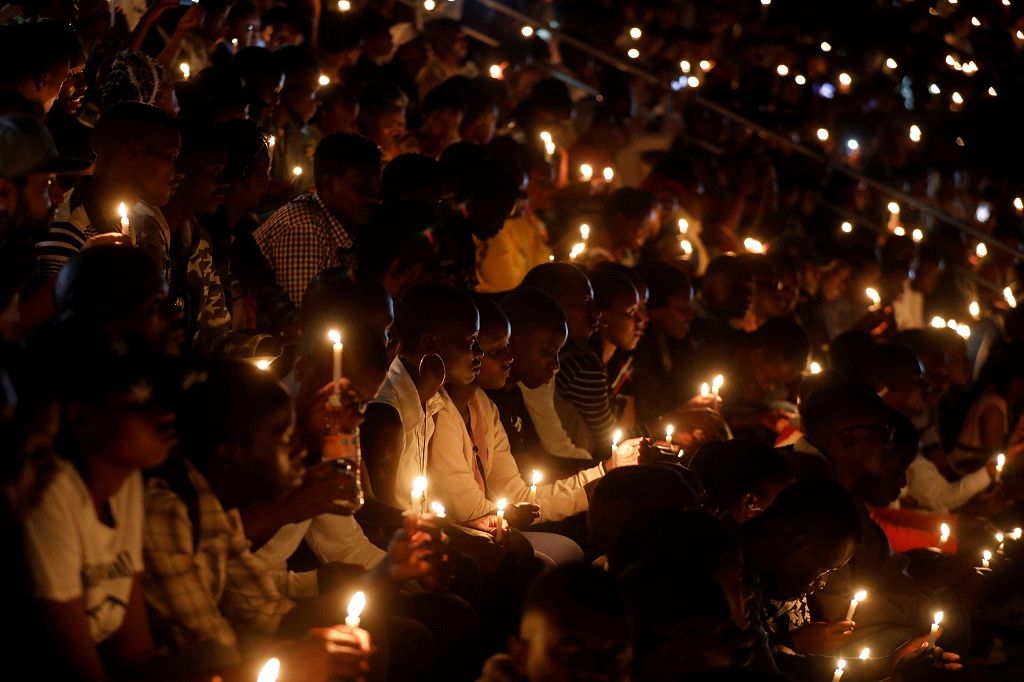The photo captures a solemn nighttime vigil with a vast crowd of African or African-American individuals, their dark skin illuminated solely by the glow of the candles they hold. The scene is filled with rows of men, women, and children seated closely side by side, their serious expressions suggesting they are either praying or mourning. The image extends far into the background, where the small flecks of candlelight merge into an expansive sea of light. Many participants are dressed in light-colored clothing, with notable garments including a child in a white t-shirt, a man with plaid long sleeves, a woman wearing a big hooped earring with a white outfit, someone in a black outfit with white stripes, and a man in a checkered shirt. The candles are simple, long stick candles, and the attendees look intently ahead, their faces partially obscured in the dim light, casting an aura of quiet reverence and unity.